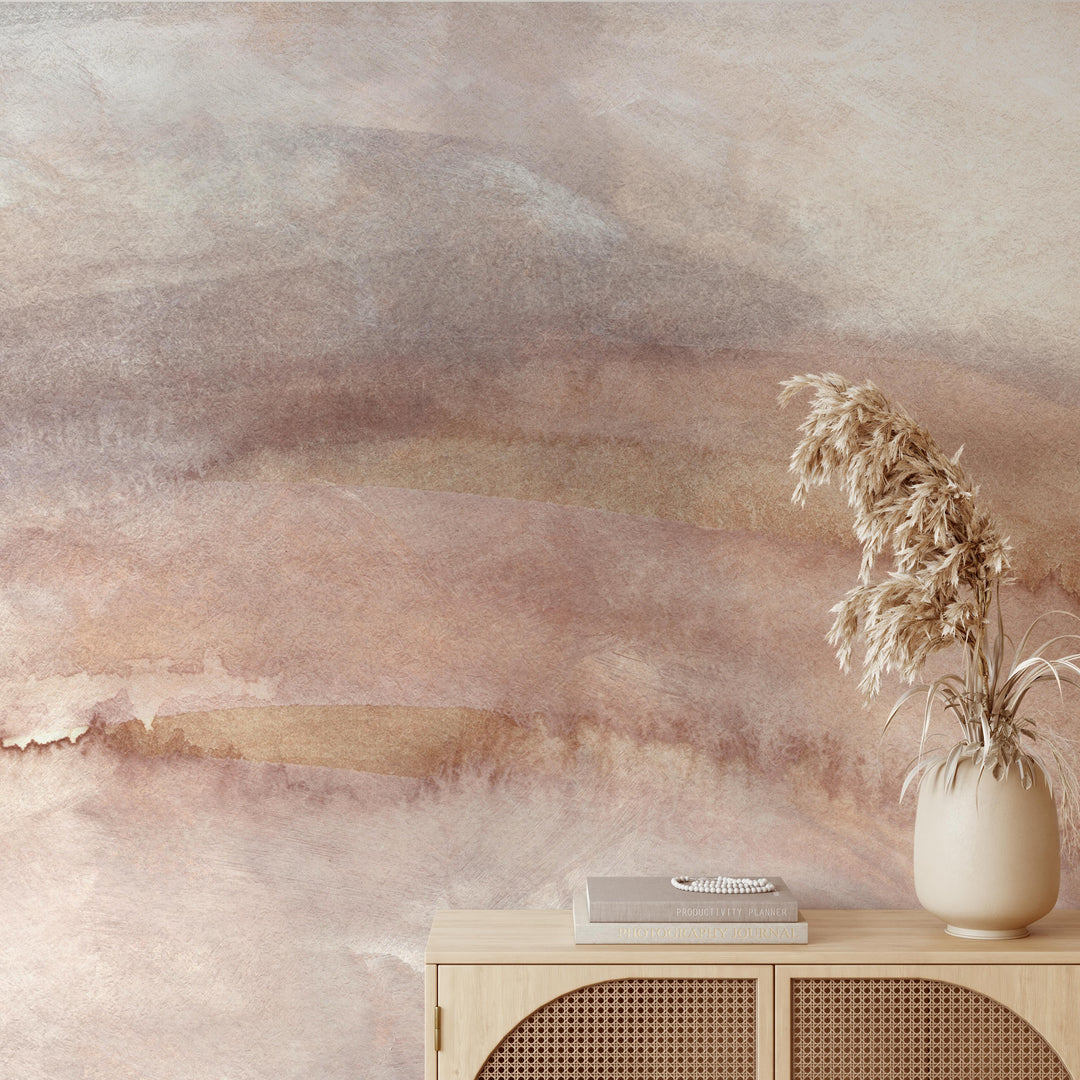A calming, faded photograph in gray and beige tones with hints of very light pink captures a tall room with a console cabinet against a softly blended, pastel-painted wall that mimics an expansive field or prairie scene. The cabinet, in a light whitish beige hue, features rattan front doors with a decorative mesh pattern. Atop the cabinet, there are two books, one in light beige and the other in shades of gray, accompanied by a strand of white beads. A simple, medium-sized vase with a light cream tan color sits next to the books, housing tall, wispy dried flowers that resemble painted wheat stalks or pompous grass in a matching faded tan cream color, along with some similarly colored leaves. The overall aesthetic of the image is very soft, cohesive, and serene, with harmonious colors and textures that give a washed-out, vintage feel.